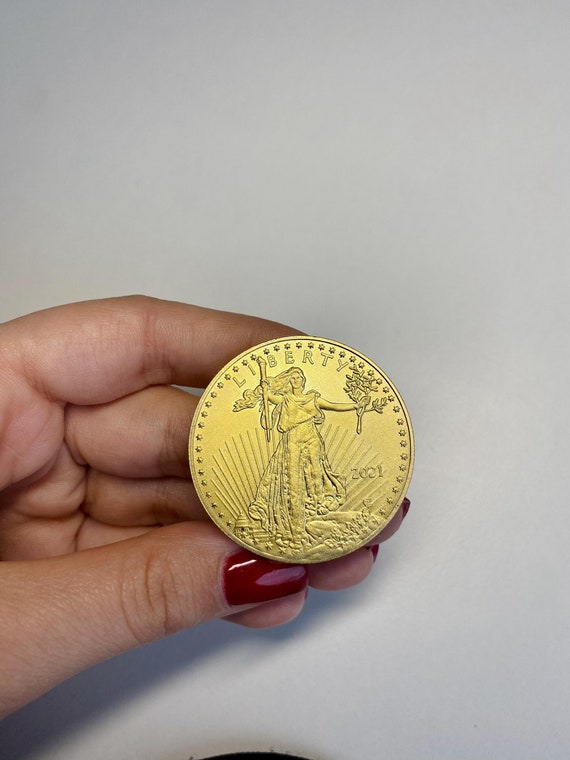In this detailed image, we see a close-up of a white woman's hand with her fingers held together, showcasing a gold coin resting on them. The woman's fingernails are neatly painted a shiny wine red color. The coin prominently features the word "Liberty" at the top, with the year "2021" marked beside it. The design on the coin includes Lady Liberty, depicted as a thin woman with long hair flowing in the wind, dressed in loose garments. She holds a torch in one hand and a branch in the other, with several stars encircling the edges of the coin. Additionally, radiant lines extend from behind her figure, enhancing the intricate detailing of the coin. A small black mark is visible at the bottom of the image, adding to the depth and authentic feel of the scene.